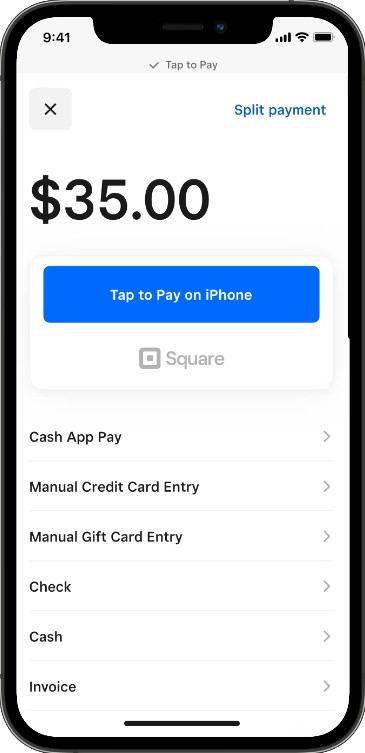The image displays a detailed view of a cell phone screen. The phone itself is outlined in black. In the upper left corner, the time is shown as 9:41 in black text. On the upper right corner, a black, fully-filled battery icon indicates a full charge.

To the right of the battery icon, there's a small gray checkmark accompanied by a "Tap to pay" prompt on the screen. Below this, on the left side, a gray square with an 'X' inside is featured. Nearby, several inches to the right, the words "Split Payment" are written in blue text.

Prominently displayed in large black text in the center of the screen is a dollar sign followed by the amount "35.00," indicating a total of $35.00. Below this, there is a horizontal blue rectangle with the text "Tap to pay on iPhone." Underneath this blue rectangle, the option to "Use Square" is written in gray text.

On the left side of the screen, a vertical list of payment method subcategories is displayed in black text. These subcategories include:
- Cash App Pay
- Manual Credit Card Entry
- Manual Gift Card Entry
- Check
- Cash
- Invoice

At the bottom of the phone screen, a black horizontal line, approximately three inches long, runs across the entirety of the phone’s lower edge, framing the detailed information described above.